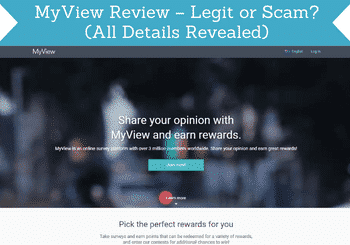**Detailed Caption**:

This is a screenshot of a home page. The top border, approximately an inch in height, is light blue and features decorative angled cuts inward from the corners, creating a clipped effect. Prominently displayed across the top in large white letters is the text: "My View Review - Legit or Scam?" Below this, in parentheses, it reads: "All details revealed." A thin gray border is positioned on the left side, while the right side features a blue section with the text "Log In," followed by some illegible text. 

Taking up most of the page below the header is a blurry image, seemingly depicting people sitting outside, but it's indistinct. Across the center of this image in bold white letters are the words: "Share your opinions with My View and earn rewards." 

Further down, there is another row of white text that's too blurry to decipher clearly. A prominent blue search bar with the words "Join Now" in white rests below this text. Directly beneath the search bar is a red circle featuring white lettering. 

The lowest portion of the page is bordered in white, featuring black text: "Pick the perfect rewards for you," followed by instructions to "Take surveys and even pose questions for a variety of rewards," though the last part is again difficult to read due to blurriness.